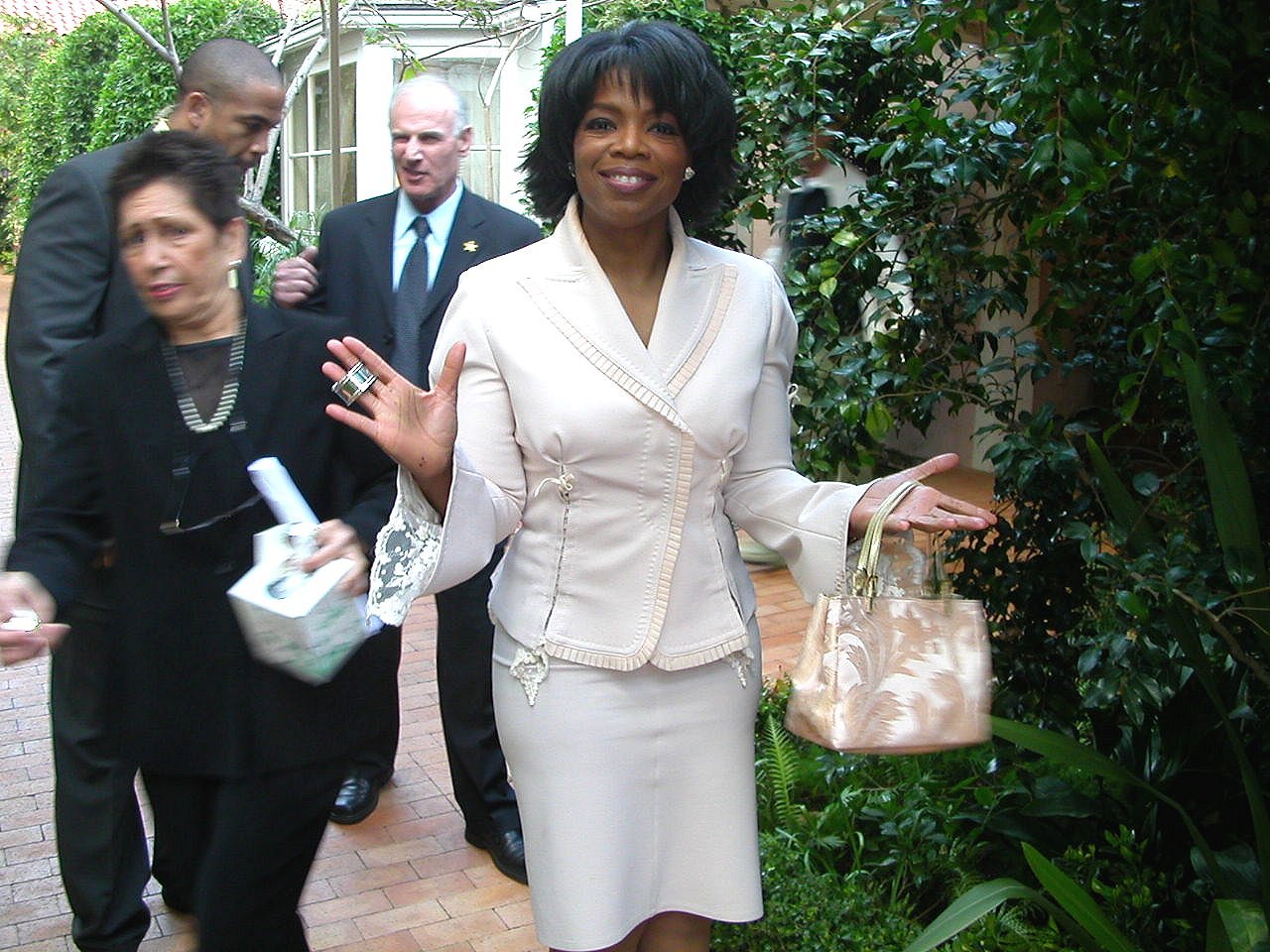The image depicts a younger Oprah Winfrey, likely in her 40s or 50s, standing in an outdoor garden courtyard area in front of a white building with visible exterior walls and windows. She is smiling warmly at the camera, with both hands raised slightly. Oprah is dressed in a stylish white leather suit comprising a white jacket and skirt, and she carries a whitish handbag adorned with beige floral designs in one hand. On her other hand, she wears a silver band around two of her middle fingers.

In the background, partially out of focus, are three individuals: a woman in a black suit with a silver necklace, holding what seems to be a box of tissues, and two men in dark blue suits, one of whom is a tall black man, and the other a shorter, older white man with white or light blue undershirts and ties. They are standing on a reddish-brick walkway surrounded by landscaped greenery, including trees, bushes, and grass. The courtyard features a lot of green leaves and plant life, making the scene lush and vibrant with a hint of a brown-roofed house in the background. In the top left corner of the image, there is a partially visible structure that looks like a cage, though its purpose is unclear.